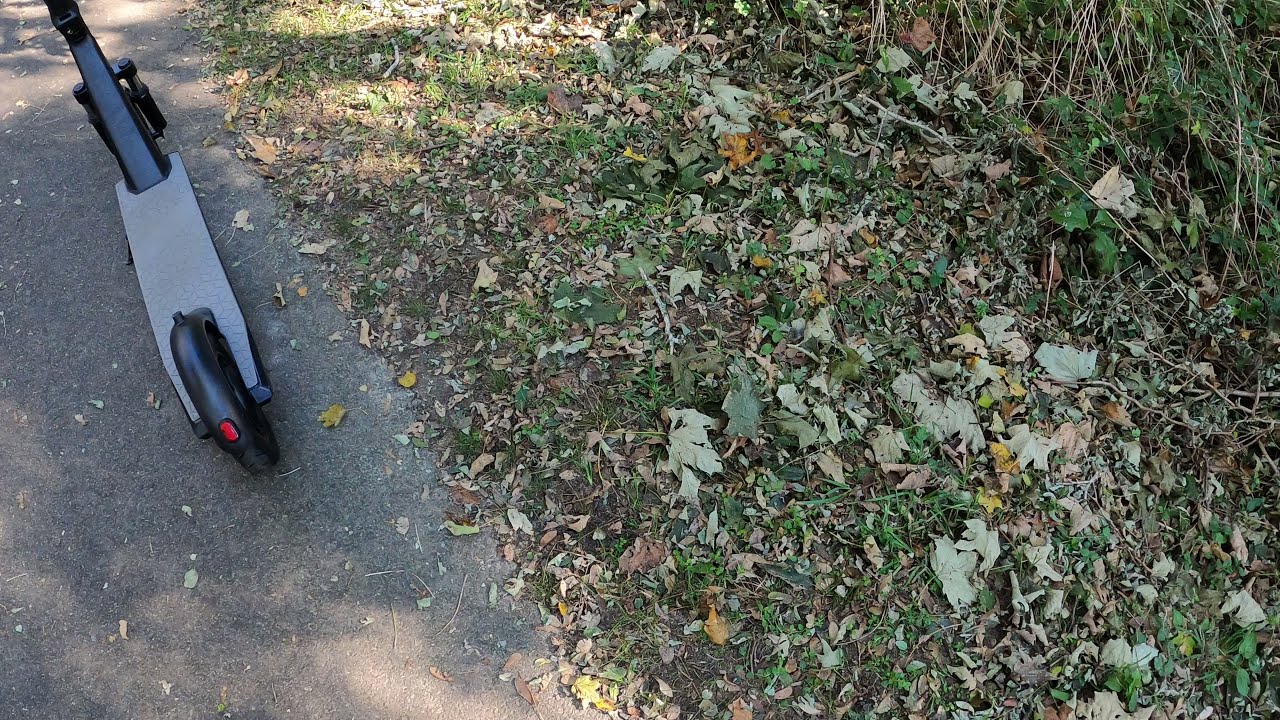The image depicts a black electric scooter parked on a dark-colored paved surface, located in the top left corner of the frame. The ground is lightly spattered with sunlight, suggesting it is daytime, likely during the summer or early autumn. The scooter features a grayish pad or footplate and shows part of the stem leading to the handlebars, which are not visible as they extend beyond the upper frame of the photograph. The left side of the image shows the edge of a road or path, while the right side of the image transitions into a grassy area surrounded by bushy underbrush and scattered leaves, indicating a natural environment with dense vegetation. The photo is taken from a slightly elevated angle, looking downwards towards the ground, providing a comprehensive view of both the scooter and its surroundings. The angle and light reflections on the grass accentuate the sunlight and the season, capturing the essence of a calm, clear day.